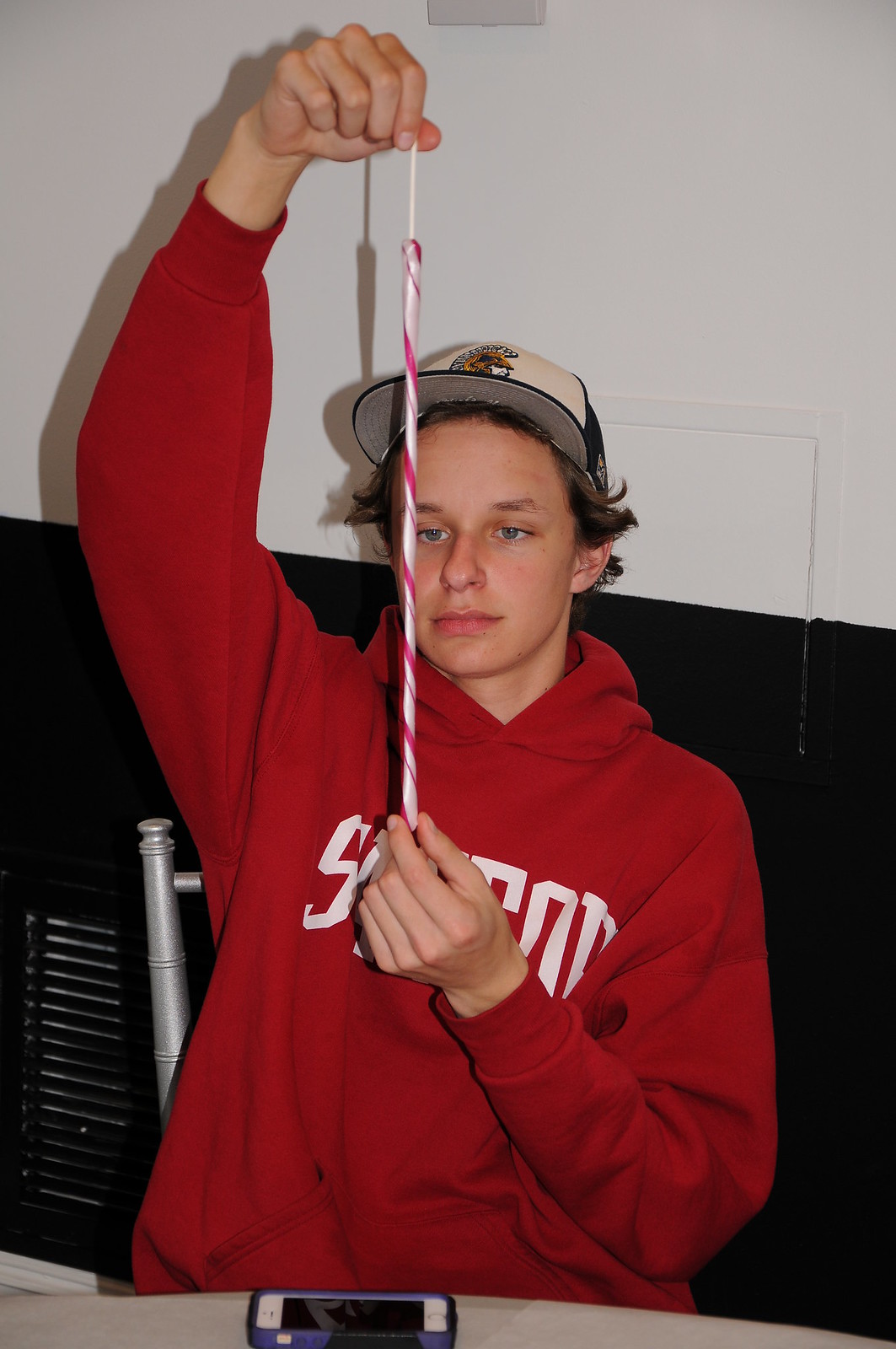In the photograph, a young man, possibly a teenager around 16 or 17 years old, is seen sitting at a white table. He is focused intently on handling a long peppermint candy stick, which he holds with both hands—one hand raising it high and the other steadying the bottom. The candy, which has diagonal red and white stripes, appears to be a work in progress, suggesting he might be crafting or stretching it. The young man is dressed in a red hoodie with white text partially obscured by the folds and his hand. Additionally, he wears a black and white baseball cap, featuring an indiscernible logo.

His bright blue eyes gaze down at the candy with concentration, and a faint smile can be seen on his face, illustrating his engagement with the task. In front of him, on the white table, lies a blue iPhone, an older model with a protective purple cover. The backdrop features a distinct two-toned wall: the upper half is white, while the lower half is black with a visible ventilation grate embedded within it. The photograph is illuminated by a flash, resulting in pronounced shadows that add depth to the image.